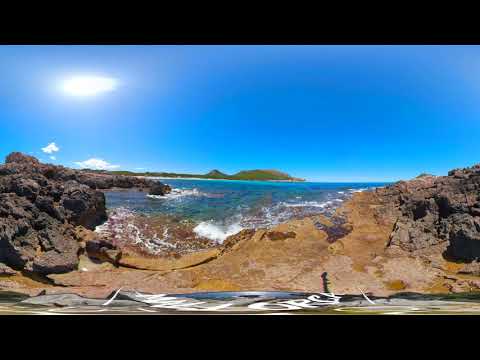The image captures a rocky shoreline with no sand, dominated by light tan rocks in the foreground and dark brown rocks stretching along the left-hand side into the water. The rocky terrain forms a U-shape, with higher rocks on the left and right that curve downwards towards the center, creating a natural trough. A narrow streak of water makes its way through the rocks, forming a small channel that spans from left to right. The dark brown rocks hook towards the background on the left and form a small mound on the right before disappearing out of view. Blue, clear water splashes against the rocks close to the shore, while the distant water remains calm. A paved area with a banner is visible at the very bottom of the image. In the distance, a landmass with a small, green hill that resembles a dolphin shape rises and falls against a backdrop of a big blue sky stippled with a few puffy clouds. The sun is shining brightly, indicating it's the middle of the day, and the weather is perfect.